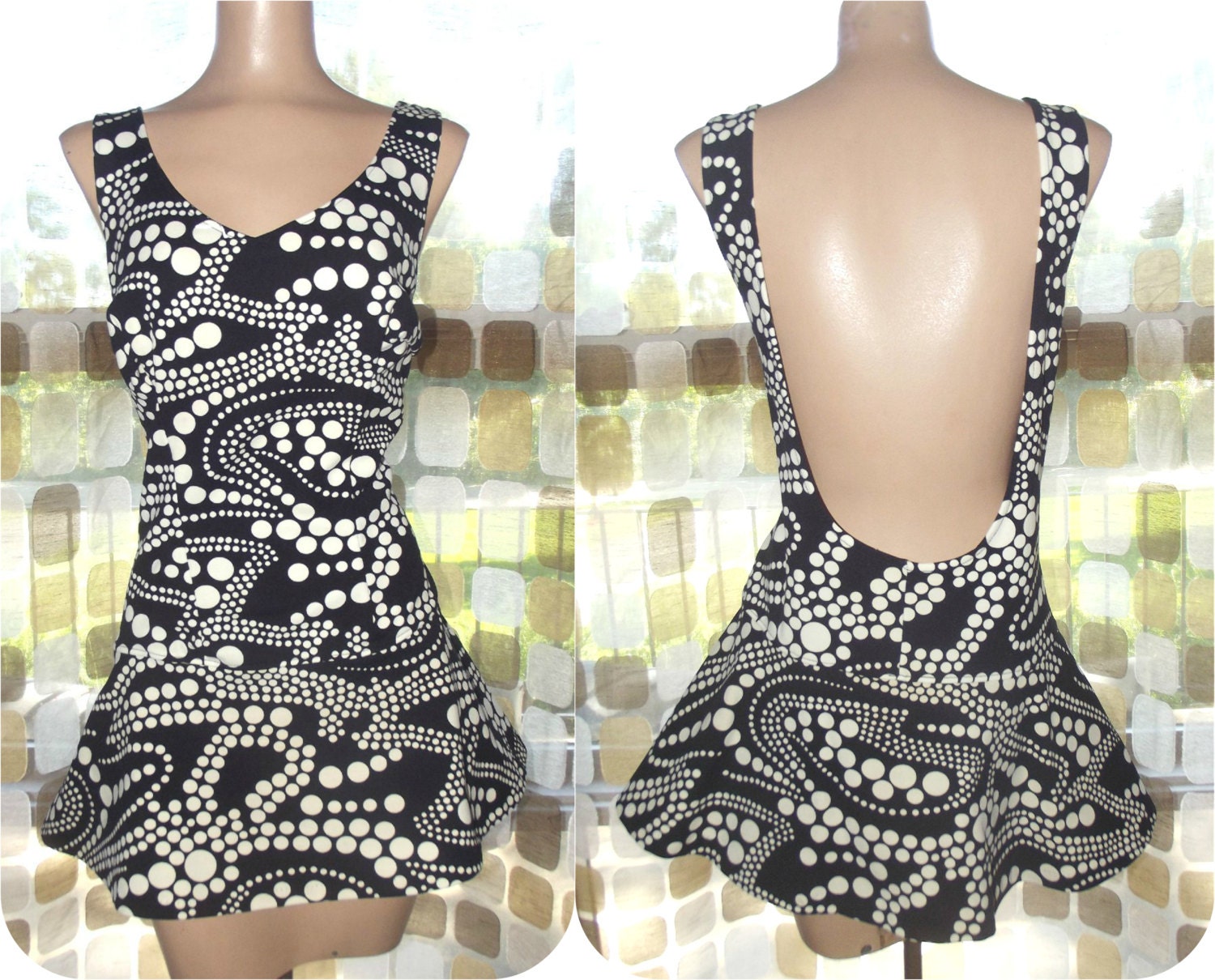This image features a side-by-side comparison of the front and back views of a feminine, headless mannequin dressed in a distinctive, summery A-line dress. The photograph appears somewhat grainy, suggesting it was likely taken with an older smartphone or digital camera. The mannequin, which is a taupe color, is positioned on a patio outdoors. 

On the left, the dress is showcased from the front, revealing a stylish black, white, and gray V-neck, sleeveless design. The fabric appears to have a unique pattern where black and white sections resemble a ribbon-like material interspersed with circular white elements on a black backdrop.

On the right, the same dress is displayed from the back, highlighting its backless feature that exposes the entire back and accentuates a flaring, short hemline. The dress's playful and breezy cut makes it ideal for summer outings. The outdoor setting on a patio further emphasizes the casual, yet chic nature of the attire.